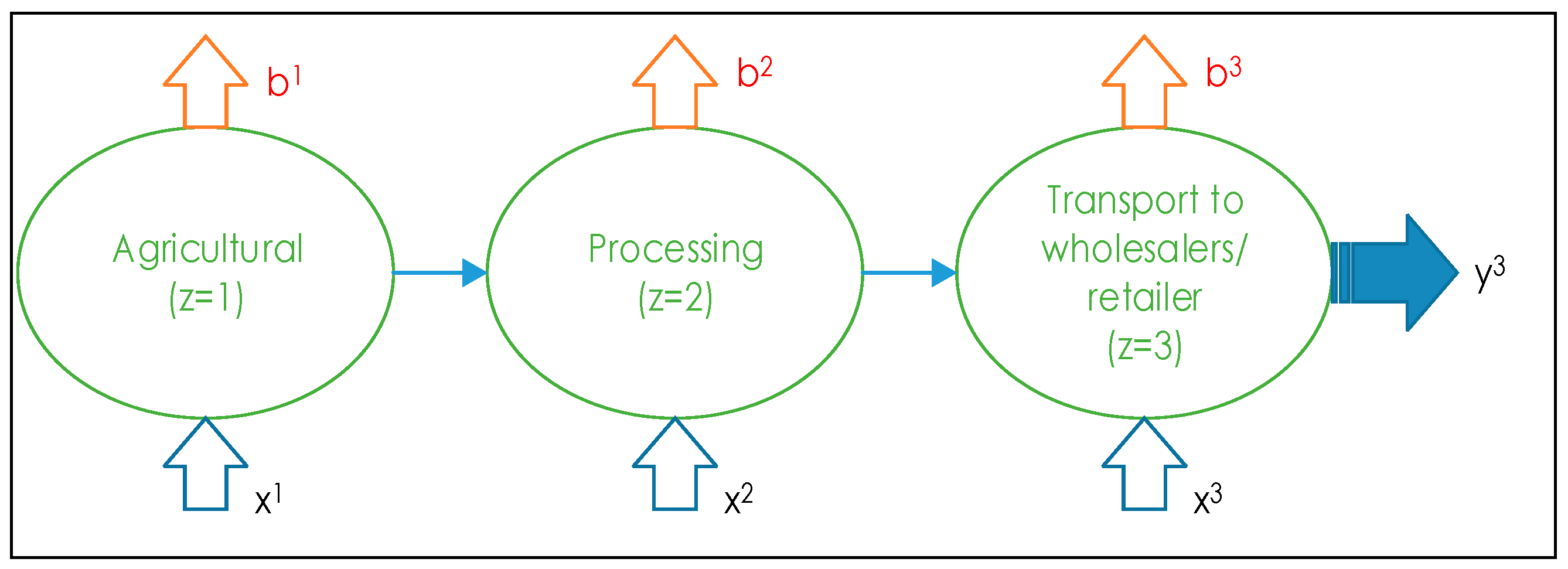The image is a rectangular infographic with a thin black border on a white background, featuring three sequential green circles in the center, each labeled and connected by lined blue arrows pointing to the right. The leftmost circle is titled "Agriculture" with a sub-label "Z = 1," the center circle is labeled "Processing" with "Z = 2" underneath, and the rightmost circle reads "Transport to Wholesalers/Retailers" with "Z = 3" beneath it. Each circle has an orange arrow above it, labeled B1, B2, and B3 respectively, pointing upwards. Below each circle is another blue lined arrow pointing upwards, marked X1, X2, and X3 accordingly. The final blue arrow exiting the last circle is thicker and filled in, directing towards "Y3." This detailed arrangement creates a clear, structured diagram likely intended for a presentation or slide, demonstrating a process flow from agriculture through processing to transportation.